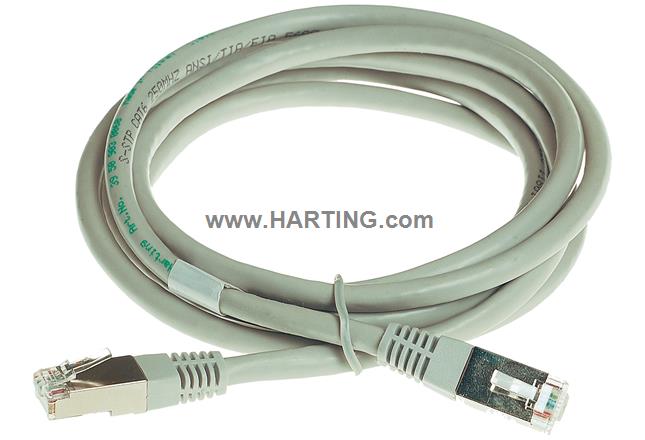This is a detailed product image of a coiled Ethernet Category 6 (Cat 6) cable, which appears to be white with a subtle whitish-gray-beige tint. The cable is tightly wound and secured with a zip tie, showcasing both ends sticking out to the left and right in the foreground, indicating the high-quality and professional splicing typical of commercial products. Prominent in the center of the image is a darker gray watermark reading "www.harding.com," likely denoting the manufacturer or distributor. The cable itself bears labeling in green and black, with legible details including "S-STP-CAT6-250MHZ-ANSI-TIA-F" along its length, emphasizing its modern 250 MHz capability. The plain white background reinforces the product-focused nature of the image, resembling those seen in online catalogs or e-commerce websites selling various types of cables.